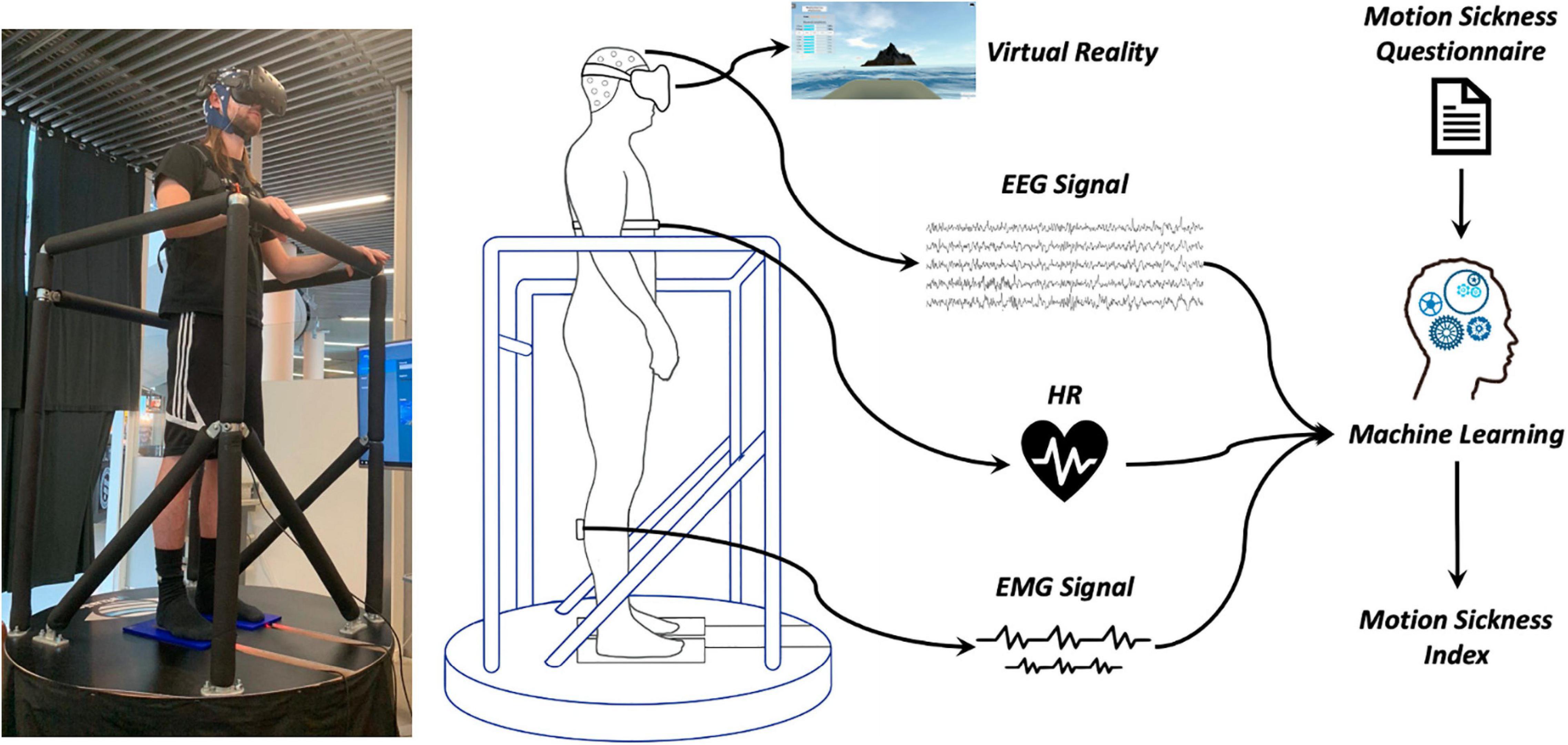The image displays a person standing on a black platform with a surrounding chest-level railing. The individual is wearing black virtual reality goggles, a black t-shirt, black shorts with white stripes, black socks, and has long hair. Positioned on the left side of the image is a photo of this person facing right, their hands resting on the railing. On the right side of the image is a detailed diagram of a similarly positioned person. 

This diagram features several annotated arrows: one arrow extends from the VR goggles to a label reading "virtual reality"; another arrow starts from the head, labeled "EEG signal" with wavy lines; a third arrow starts from the chest with "HR" indicating heart rate; and the last arrow from the back of the leg is marked "EMG signal." All these signals converge into a single arrow leading to a profile image of a head with gears, labeled "machine learning." Above these arrows, the diagram is labeled "motion sickness questionnaire," and below, it reads "motion sickness index."